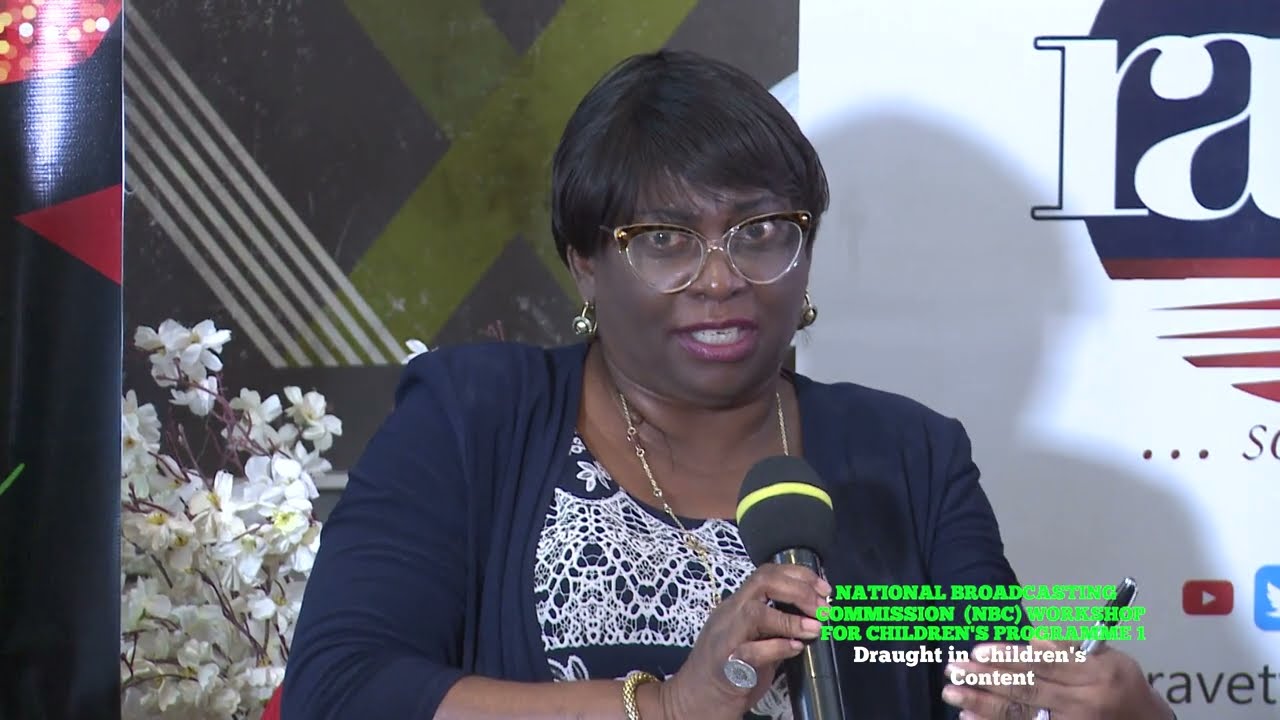The image is a rectangular photograph featuring an African American woman, likely in her early 40s, standing and holding a microphone in her right hand as if mid-speech. She's wearing distinctive cat-eye glasses with brown frames that are clear at the bottoms. Her short, dark hair just reaches the top of her neck. The woman is dressed in a navy blue blazer over a navy and white patterned blouse or dress, accompanied by earrings and a necklace. You can also see that she wears a bracelet and two rings on her right hand, and another ring on her left hand which is holding a pen. Behind her, various signs suggest it's a formal event, with backgrounds ranging from black and red to green and brown, including white flowers visible over her shoulder. At the bottom right of the photograph, the text "National Broadcasting Commission NBC Workshop for Children's Program 1" is superimposed in bright green, with "Drought in Children's Content" in white below it, indicating the event is likely a seminar on children's programming challenges.